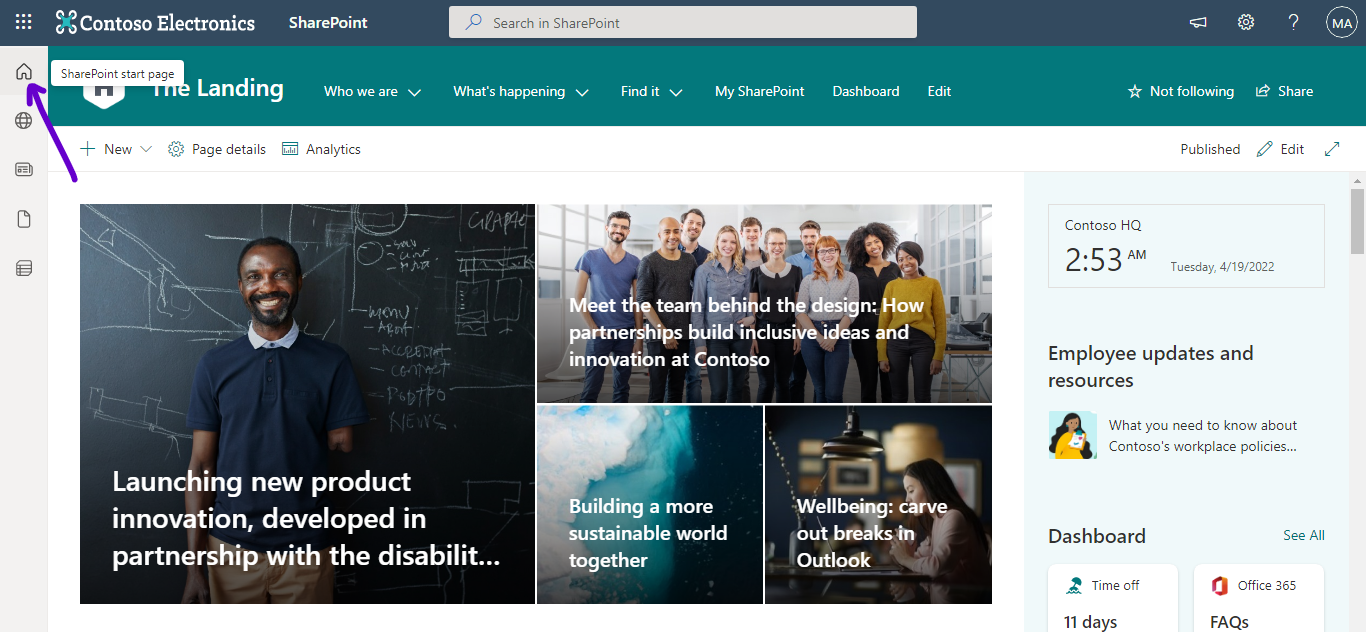On the Contoso Electronics SharePoint landing page, the website's layout is as follows:

- **Header Section**: The Contoso Electronics logo is positioned on the left side, with the SharePoint logo and a search bar adjacent to it. To the right, there are icons for settings (depicted by a gear wheel), a help section (represented by a question mark), and user initials "MA."

- **Left Sidebar**: The vertical navigation column consists of a home button at the top, followed by a globe icon, and three additional icons which are not clearly identifiable but possibly represent a copy function, a map, or a calendar.

- **Main Content Area**: 
  - **Navigation Menus**: This includes the SharePoint start page marker, emphasized with a purple arrow. Below this are expandable sections titled "The Landing," "Who We Are" (with a drop-down arrow), "What's Happening" (drop-down arrow), "Find It" (drop-down arrow), and "My SharePoint," followed by links to the "Dashboard" and "Edit" options. A star icon indicating “Not Following” and a share icon are also present.
  - **Highlighted Articles**: 
    - **Primary Article**: An image portrays an educator in front of a chalkboard filled with scientific or mathematical illustrations. The article is titled "Launching New Product Innovation Developed in Partnership with the Disability."
    - **Secondary Article**: Titled "Meet the Team Behind the Design: How Partnerships Build Inclusive Ideas and Innovation at Contoso," it features images of ten team members: five women (comprising two African American and three European descent) and five men (all of European descent).
    - **Additional Articles**: "Building a More Sustainable World Together," focusing on sustainability, and "Well-being Carve Out Breaks and Outlook," addressing wellness tips.
  
- **Footer Content**: Displays timestamp and location information: Contoso HQ, 2:53 a.m., Tuesday, April 19, 2022. It also includes sections like "Employee Updates and Resources," detailing workplace policies, and "Dashboard Time Off," indicating 11 days available, along with links to "Office 365" and "FAQs."

- **User Actions**: Options for creating new content (button labeled "+ New" with a drop-down arrow), and icons for "Page Details," "Analytics," and editing (pencil icon).

This comprehensive layout of the Contoso Electronics SharePoint page ensures easy navigation and information accessibility for employees.